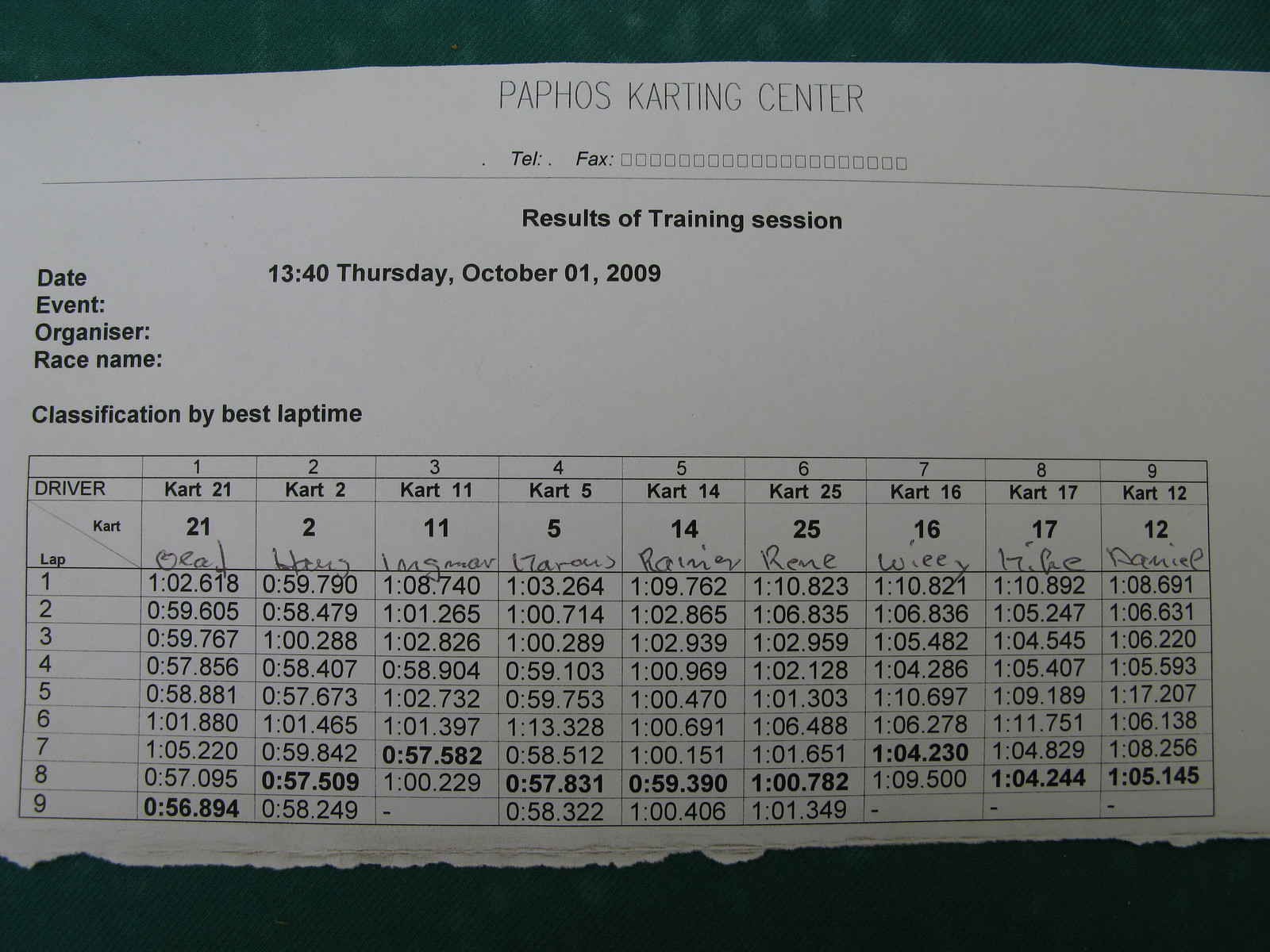This image features a piece of white paper placed against a dark background. The bottom edge of the paper is torn. The header reads "Paphos Carding Center PAPHOS" in black text, followed by "tell and fax" without any numbers. The document details the results of a training session dated "Thursday, October 1, 2009." Several fields, including "event organizer," "race name," and "classification by best lap time," are left blank. Below, a chart spans the page, with columns labeled "driver" and "lap 1" through "lap 9," followed by "cart 21," "cart 2," "cart 11," "cart 5," "cart 14," "cart 25," "cart 16," "cart 17," and "cart 12." The names of drivers, such as Renee, Willie, Mike, and Daniel, are handwritten beneath these columns, though some names are illegible. The chart records the lap times for each driver, meticulously detailing the performance metrics from their runs.